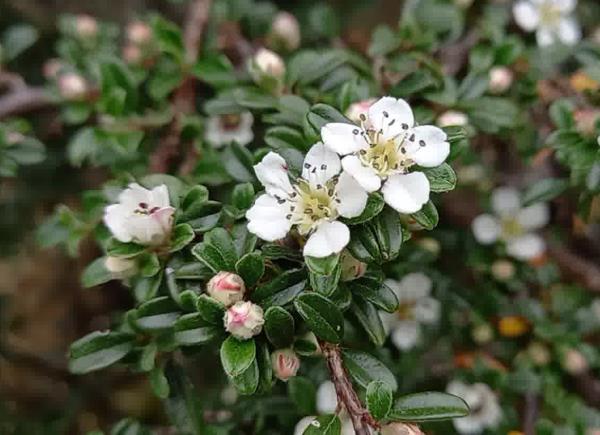This landscape-oriented close-up photograph showcases a natural grouping of white flowers, likely tulips, centered in the image. The prominent flowers each possess five rounded white petals, with a vibrant yellow core featuring thin, stringy filaments or stamen, some bearing black tips and tiny green components possibly resembling seeds. These flowers are part of a bush, evident by the shiny brown stems that curve gracefully, and the dark green, waxy, oval-shaped leaves. Surrounding these central blooms, the background is artistically blurred, revealing additional green plants and flowers at various stages of blooming. Several unopened buds, tinged with pink, are visible just below and to the left of the main flowers. The top right and lower left of the photograph are filled with a soft, verdant blur, hinting at more foliage and the natural proliferation of the floral bush.